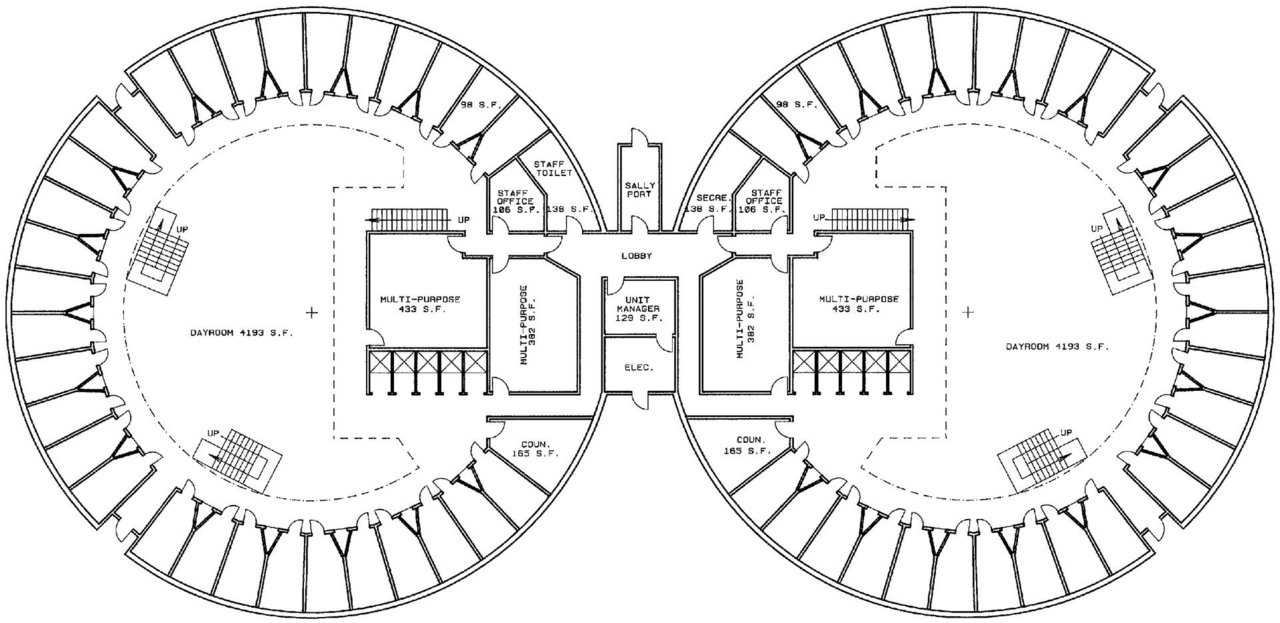This image depicts a detailed architectural blueprint of a building with two large, connected circular structures. Each circle is divided into various labeled sections by lines extending from the periphery towards the center, likely representing rooms or pathways. The left circle prominently features a "Day Room" occupying 4193 square feet, with a smaller adjacent "Multipurpose" area of 433 square feet. Additional labeled areas within the circle include a "Staff Office," "Staff Toilet," and a partially readable "C-O-U-N," which may indicate a counseling room. The central connecting structure, functioning as a lobby, includes spaces designated for a "Unit Manager," "Lobby," "Electricity," and a "Sally Port." The right circle mirrors the layout of the left, with labels for a "Day Room" and multiple "Multipurpose" areas, as well as a "Secretary," "Staff Office," and another "C-O-U-N." The entire plan is symmetrical and presented on a white background with black font, embodying a clear and precise design ethos.